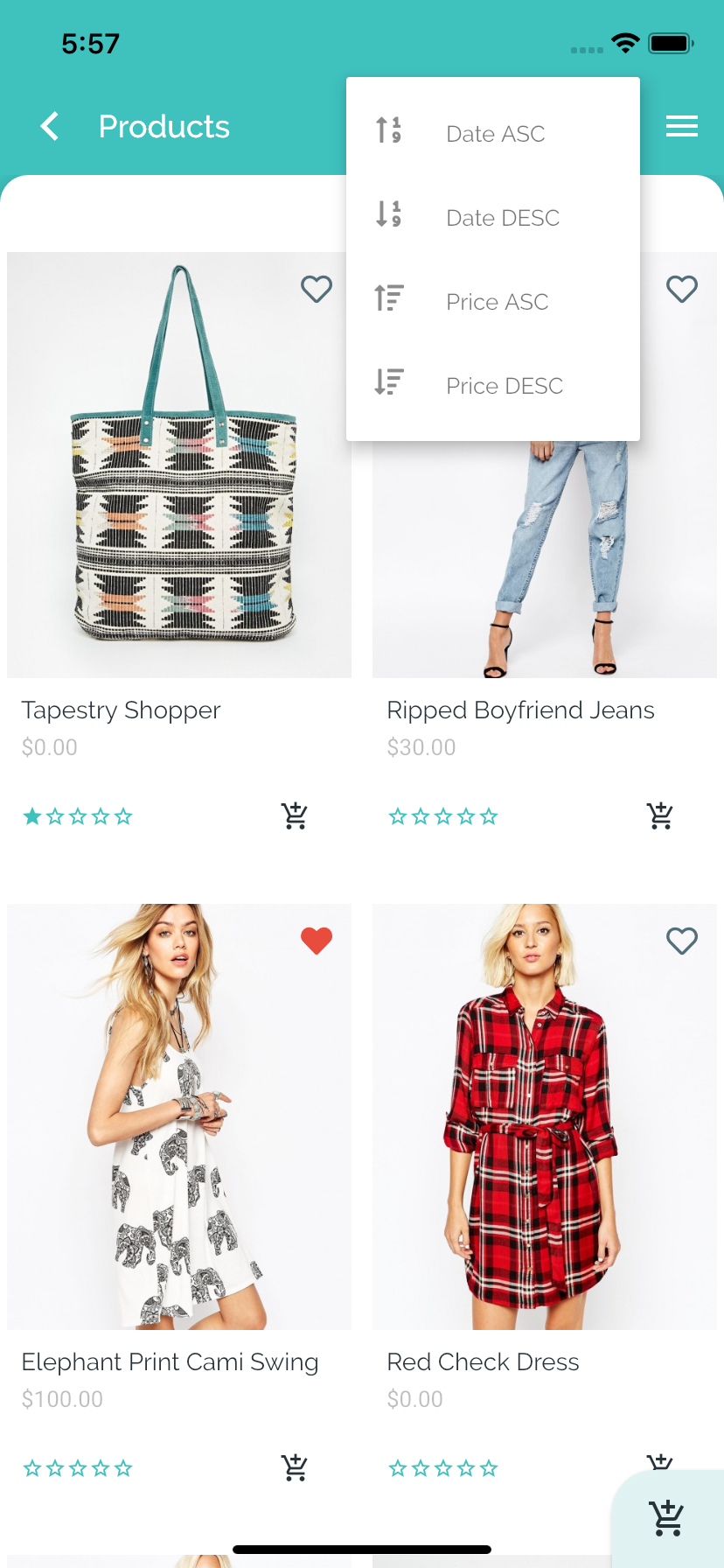This image is a screenshot of a shopping application interface, presenting various product options for purchase. At the top of the screen, a green bar displays the title "Products." Below this, the interface is divided into two rows, each featuring two product images.

In the top row, the left image showcases a bag labeled "Tapestry Shopper," and to its right, another image highlights a woman wearing "Ripped Boyfriend Jeans." The jeans picture is partially obscured by an open menu. This menu, overlaid across the top of the screen, presents sorting options: "Date ASC," "Date DESC," "Price ASC," and "Price DESC."

The bottom row contains two more product photos of women modeling clothing items. The left image features an "Elephant Print Cami Swing," distinguished by a red heart icon indicating it has been marked as a favorite. The right image displays a "Red Check Dress."

Additional interface elements include a shopping cart icon located in the bottom right-hand corner and a three-bar (hamburger) menu, Wi-Fi symbol, and battery indicator positioned at the top of the screen.